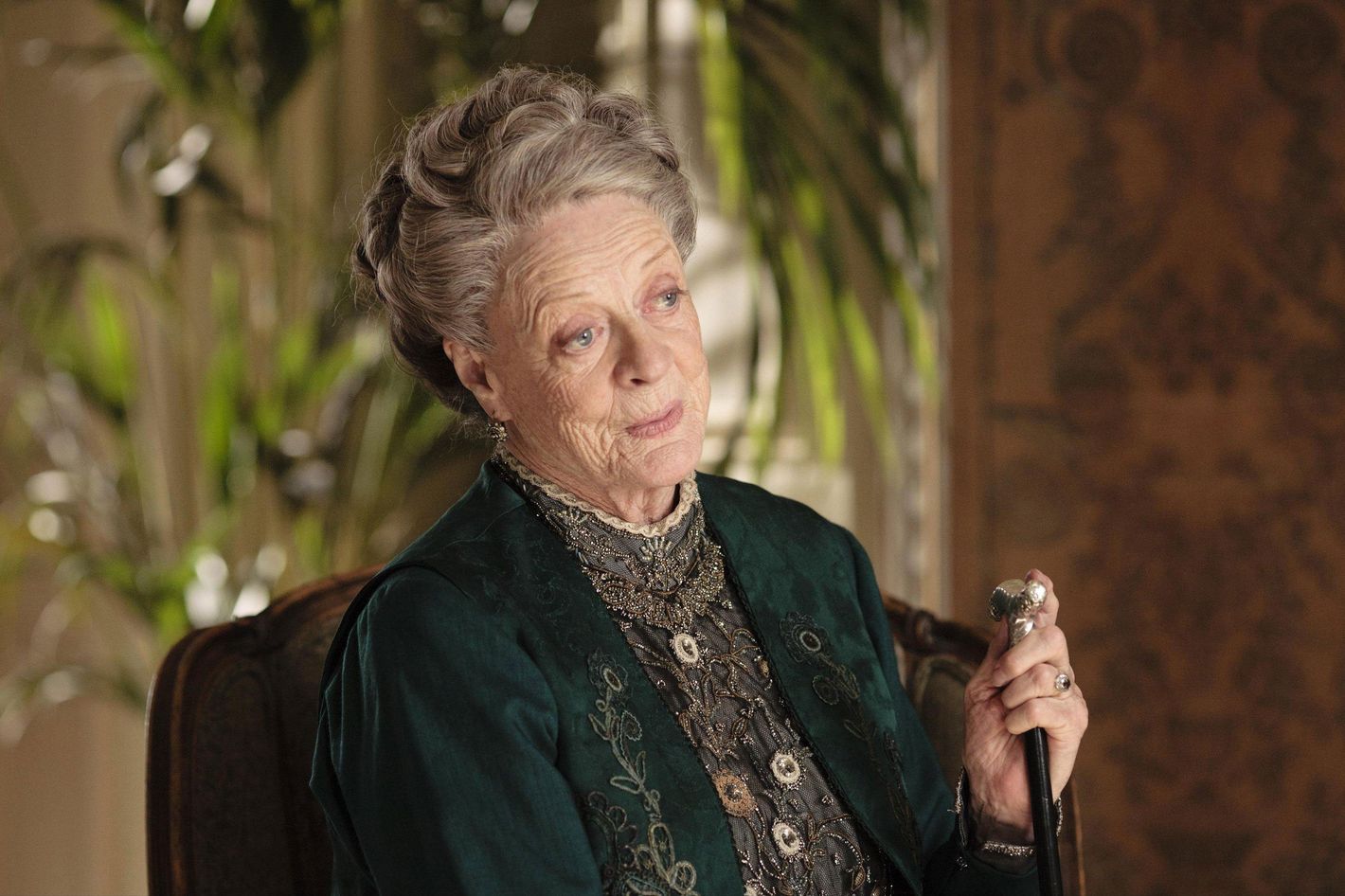In this photograph, Maggie Smith is captured in character as she role-plays in 'Downton Abbey.' She sits gracefully on a brown upholstered chair with a carved wooden frame. Behind her, a lush potted fern contrasts against rich brown damask-style wallpaper, giving the scene a historically opulent atmosphere. Maggie Smith's hair is styled in an elaborate updo, complementing her period costume. She is dressed in a teal waistcoat, embroidered on the front, worn over an elegant gray gown. The high-collared dress is richly adorned with sequins and beading, featuring intricate gray and ivory ornamentation. In her left hand, she holds a black walking stick topped with an ornamental silver knob, adding a touch of regality to her poised demeanor.